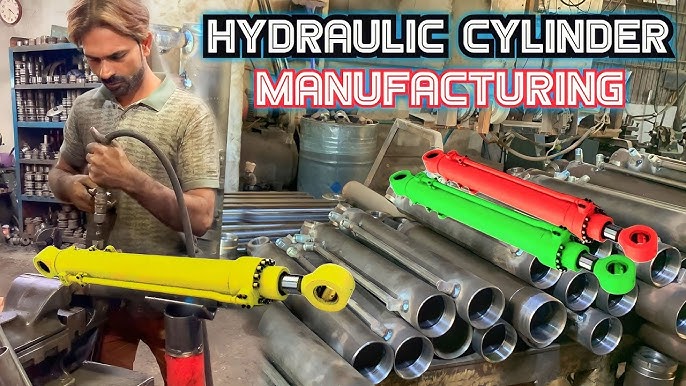A vibrant color photographic image captures the bustling environment of a hydraulic cylinder manufacturing workshop, designed to serve as an eye-catching social media video thumbnail or advertisement. In the foreground, white text with a black border and a neon glow announces "Hydraulic Cylinder Manufacturing." To the left, a young man, approximately 30 years old, focuses intently on his task. He is attired in a grey polo shirt with brown accents and shorts, with his hands busy operating a tool attached to a large yellow hydraulic cylinder secured in a workbench vise. The man appears worn but dedicated, indicative of a labor-intensive setting.

In the background, a blue metal shelf brims with machine parts, alongside a visible clock on the upper left. To the immediate left of the man, two fully assembled hydraulic cylinders—one green, one red—stand prominently, while an array of unfinished, silver metal cylinders is neatly stacked below. The workshop is vividly industrial with shelves filled with various parts, large tanks, or oil drums and an abundance of wires and metal components, painting a comprehensive picture of the manufacturing process in action.